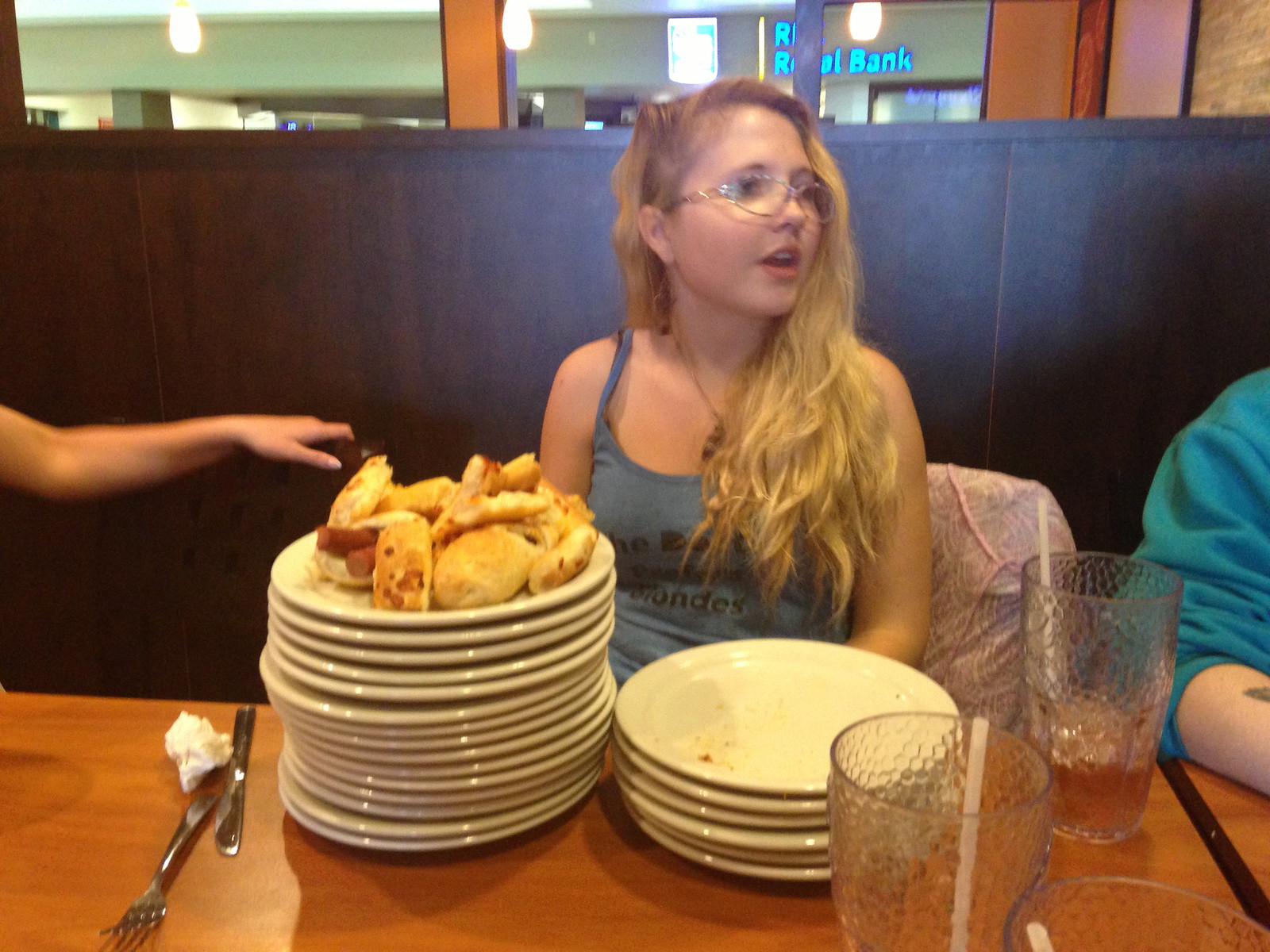In this candid photograph taken at a restaurant within what appears to be a shopping center, a young blonde-haired woman with glasses and shoulder-length hair is captured. She is seated at a light-colored wooden table with a tall, dark wooden backrest, wearing a blue tank top featuring unreadable text. In front of her, there is a towering stack of approximately 15 to 20 plates topped with several pieces of bread, including one with two sausage pieces. Additionally, a smaller stack of about seven to ten plates sits nearby, surrounded by silverware, a crumpled napkin, and three plastic drinking glasses with ice and straws, some partly filled with juice. On the left side of the image, part of a bare arm and hand are visible, while the right side includes an arm clad in a blue shirt. The backdrop features a storefront sign with the word "bank" in blue letters, hinting at the location within a commercial center. The young woman gazes off to the right, seemingly distracted by something outside the frame, giving the photo its candid and spontaneous feel.